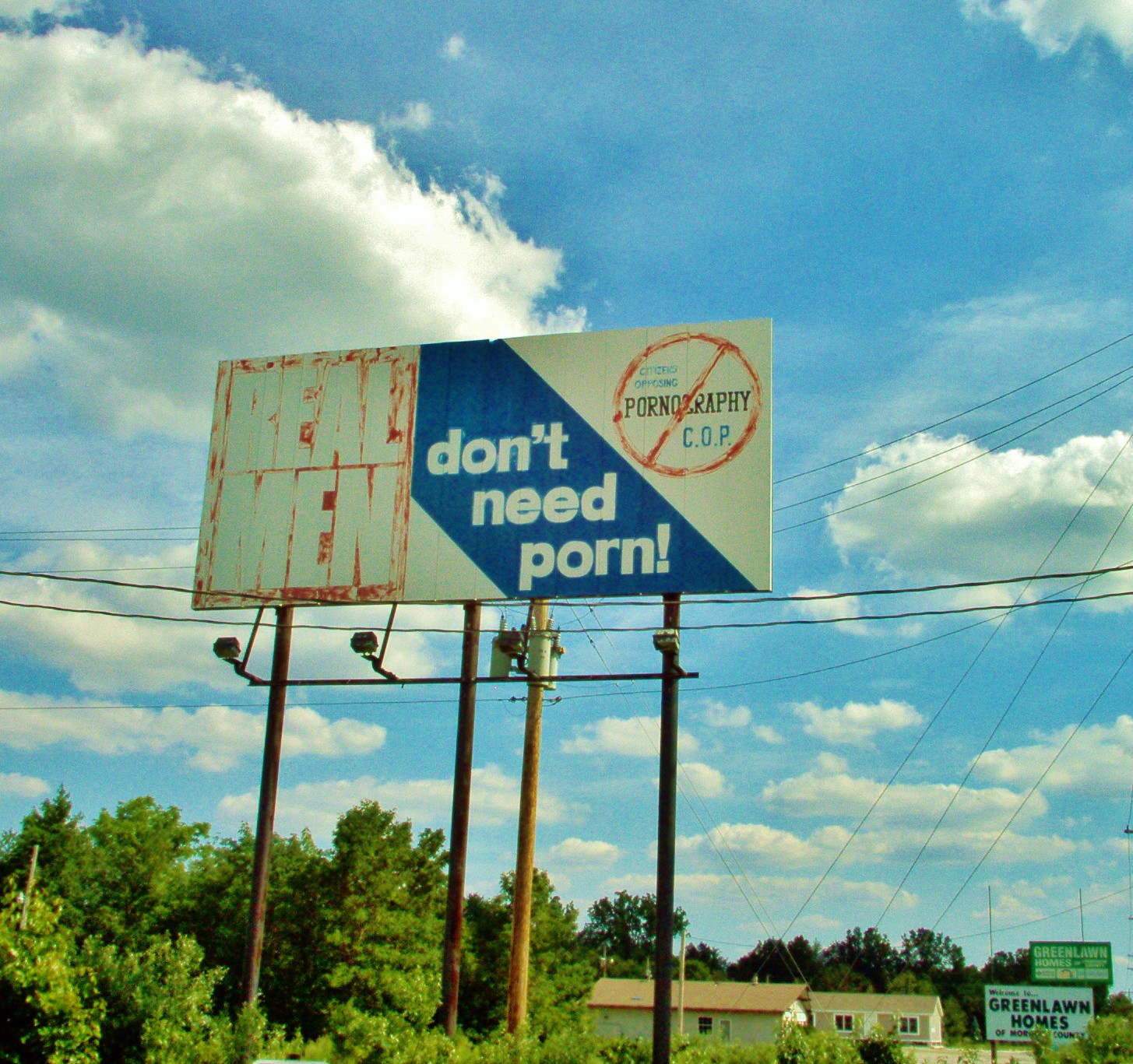This image features a weathered billboard standing tall in a wooded area. The left third of the sign boasts the message "Real Men" in large, bold white block letters set against a bright red background. The remaining two-thirds of the billboard transitions to a white backdrop, displaying a diagonal blue banner with the words "Don't Need Porn." This part of the banner is further emphasized by a prominent red "no" symbol slashing across the word "pornography," reinforcing its message. Positioned high above the trees, the billboard appears illuminated by four lights designed to flash upon it. The entire scene is set against a picturesque backdrop of a clear blue sky dotted with fluffy white clouds. Below the billboard, there are modest modular homes or single-wide trailers scattered in the green, scruffy landscape. Additionally, there's a sign indicating "Green Lawn Homes" nearby, integrating into this rustic setting.